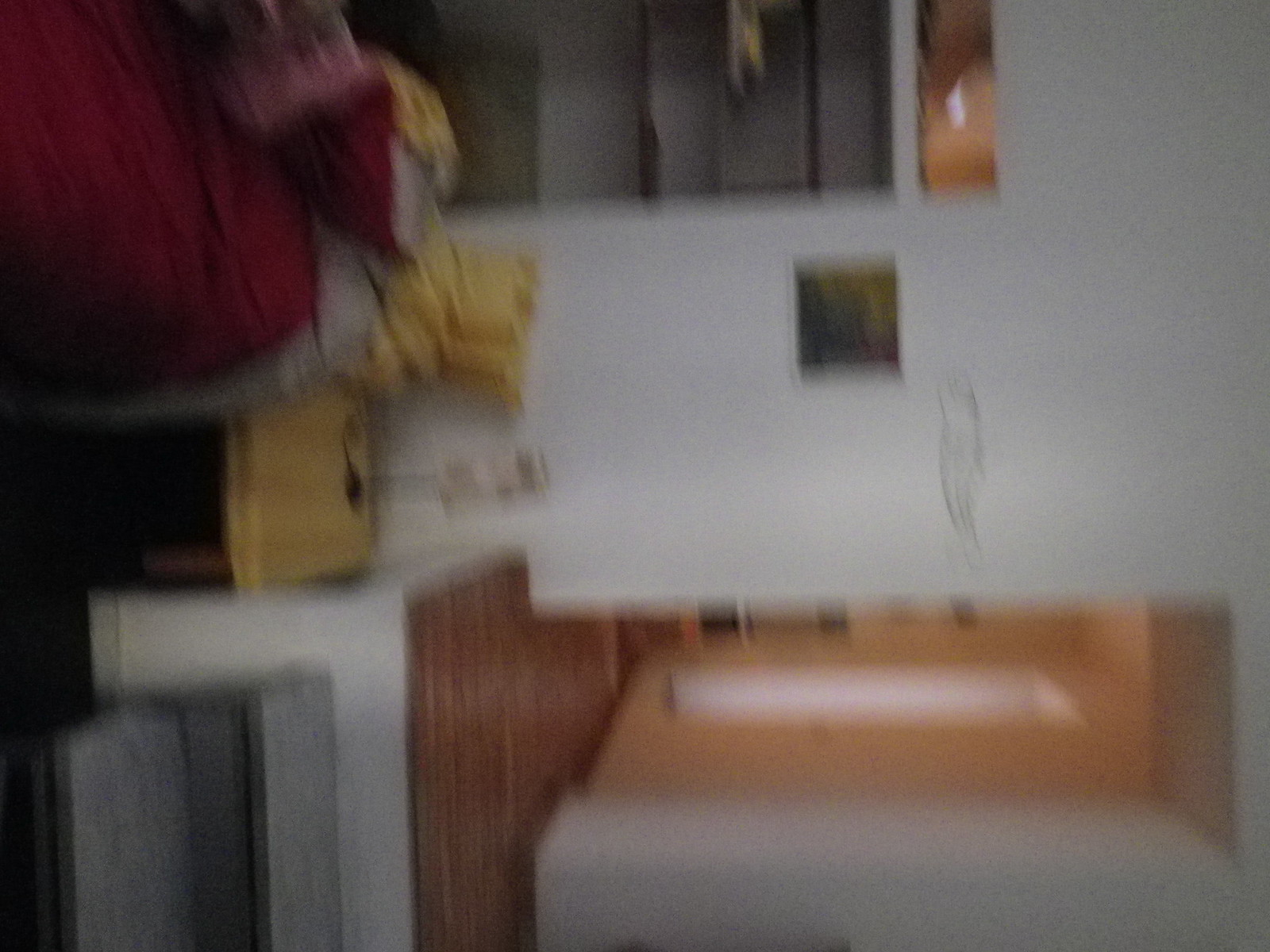The photograph is a highly blurred image of an interior space, possibly a home, apartment, or house. The image is so out of focus that definitive details are challenging to discern. A white wall is visible, adorned with rectangular and square shapes that could be wall art, mirrors, or calendars. Towards the bottom of the photo, there is an indistinct wooden structure, likely the edge of a cabinet, upon which are items that might be backpacks or blankets, distinctly colored in red and yellow. Due to the extreme blurriness, identifying specific objects or text is not feasible.